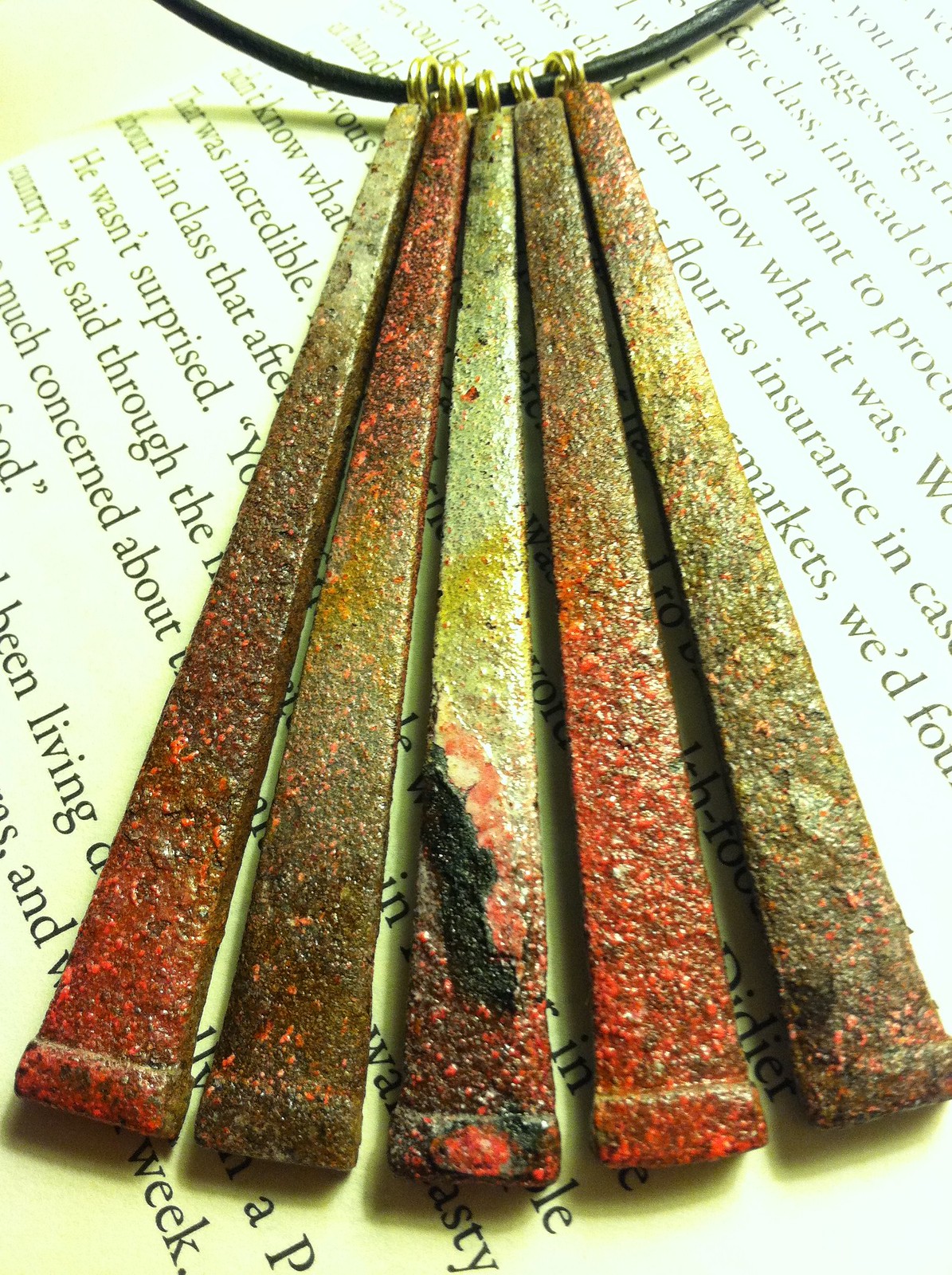The image depicts an intriguing necklace laying on the open pages of a book filled with text. The necklace features five elongated, carved stones that closely resemble rough, corroded flat nails in shape. These slender rectangular stones start thinner at the top and widen toward the bottom, reminiscent of the shape of French fries. They exhibit a rich palette of colors, including shades of rust, red, brown, yellow, beige, and black, indicating age and wear, and giving them a textured, rustic appearance. Each of these stones is suspended from a black string or wire that arches gracefully from the upper left to the upper right of the image, creating a captivating visual arc. The black string suggests a sense of structure and coherence amidst the seemingly ancient and weathered stone fragments that hang beneath it.